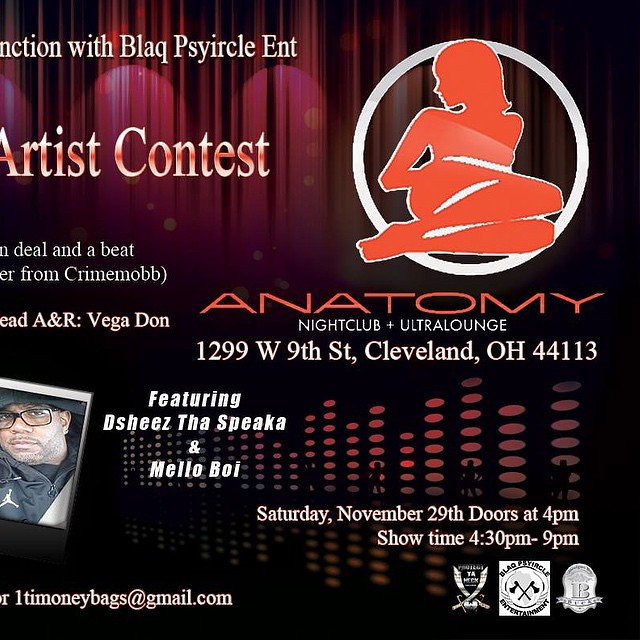This poster is an advertisement for an artist contest and event at Anatomy Nightclub and Ultra Lounge, located at 1299 West 9th Street, Cleveland, Ohio, 44113. The flyer features a wavy red and black background with a depiction of a red-colored woman with a white outline lounging within a white circle in the top right corner. In bold red letters, it prominently displays "Anatomy" and beneath, in white letters, it reads "Nightclub and Ultra Lounge." The event, scheduled for Saturday, November 29th, features performances by Dee Shees, The Speakah, and Mellow Boy. Doors open at 4 PM, and the show runs from 4:30 PM to 9 PM. The bottom of the poster lists an email address, onetimanybags@gmail.com. Additionally, there is a photograph of an African American man wearing glasses, who is possibly one of the performers. There is also mention of the rap group Prime Mob in association with an artist contest, though this part of the flyer appears partially clipped.